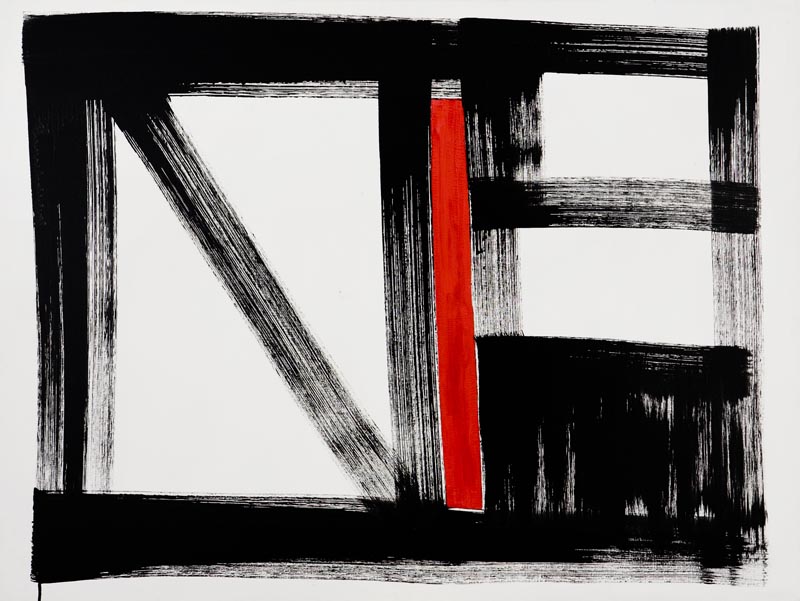This rectangular abstract painting features a series of black windows framed against a bright red rectangular section. The dominant left window includes a bold, diagonal streak that runs from the top left-hand corner to the bottom right, resembling the letter 'N.' The expressive black stroke appears textured and irregular, as if drawn with a worn-out sharpie. Adjacent to this window, a vivid red vertical stripe divides the canvas, standing slightly off-center to the right.

To the right of this red stripe is another rectangular window with a central horizontal beam splitting it midway, from the left to the right. This window also features a darker, almost black lower pane, again with a textured, streaky appearance. The entire painting has dark black outlines adding to the structural feel of the composition. The contrast between the aggressive black lines and the bold red stripe creates a striking visual tension. The absence of text allows the viewer to focus on the dynamic interplay of color and form in this expertly balanced piece of abstract art.